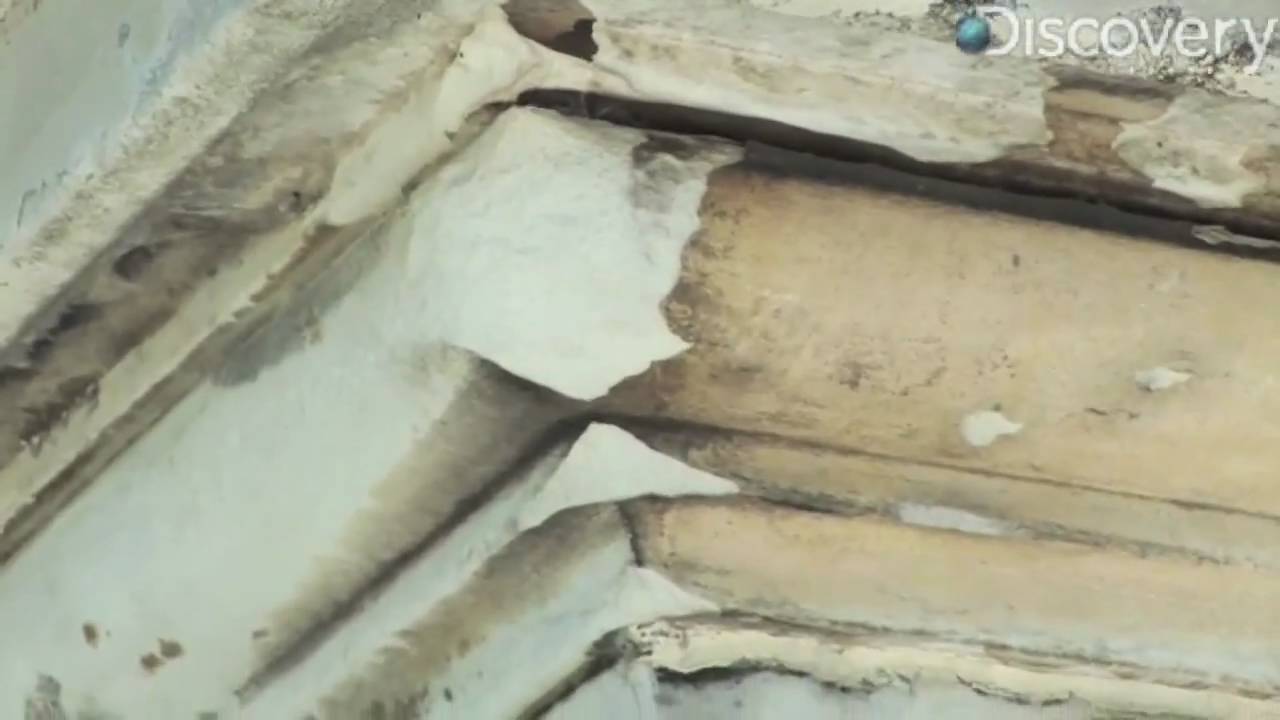This color horizontal photograph captures a close-up view of the corner of a log cabin, showcasing the intricate wood texture of the light brown logs adorned with dark mildew spots. Snow and ice have accumulated prominently on the upper left corner and more sparingly on the upper right corner, with some wood peeking through. The overall condition of the wood appears dilapidated, with remnants of white paint faded away, revealing a beige color underneath. The image hints at years of weathering, possibly with some chipping plaster or paint and potential cobwebs in the corners, suggesting neglect. A watermark featuring the Discovery Channel logo, including a small Earth globe and the word "Discovery," is visible at the top of the image, hinting that this is likely a professional photograph or screenshot from a Discovery Channel program. Shadows cast by the structure emphasize the depth and layers of the corner, adding to the detailed and textured view of this rustic scene.